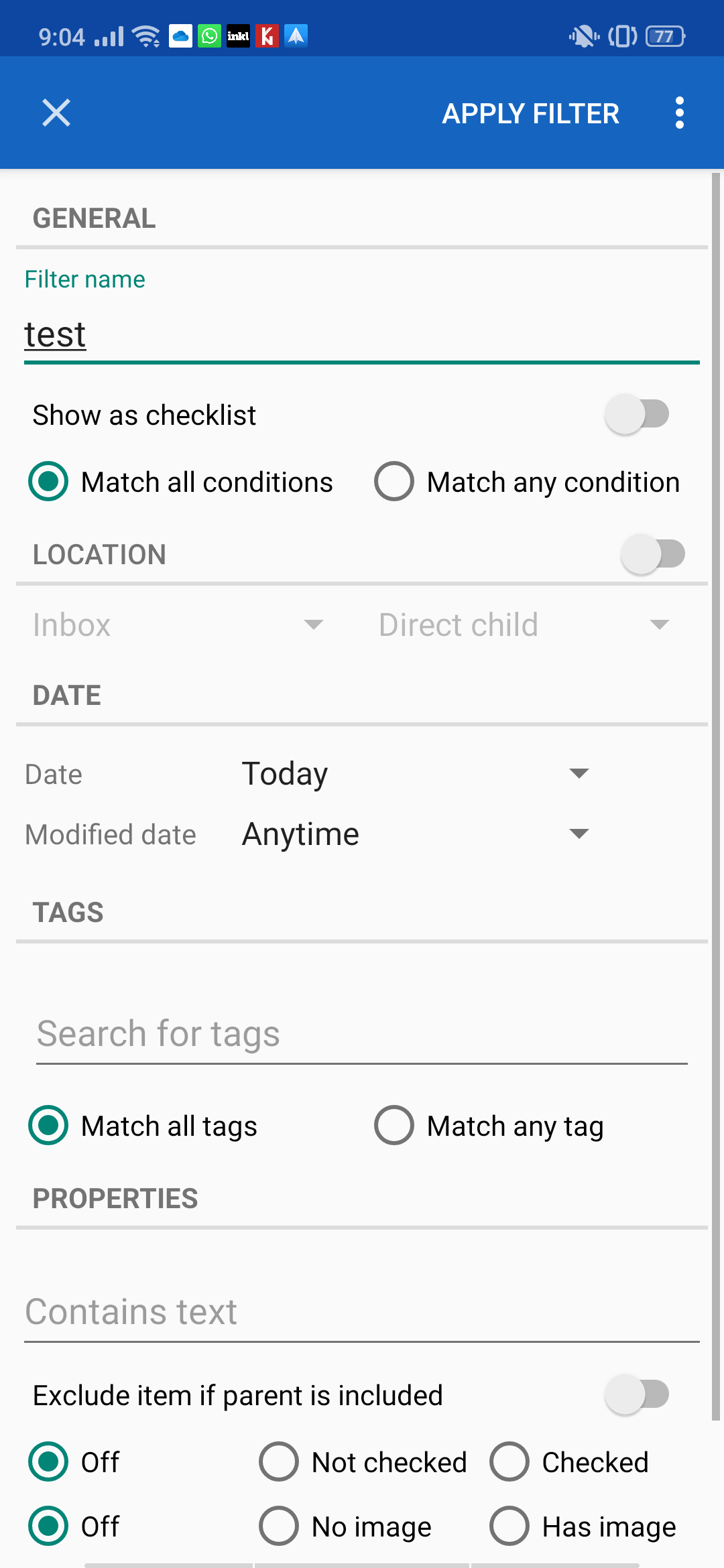This image is a screenshot displaying a user interface for applying filters, captured at 9:04 AM, with a full Wi-Fi signal and a fully charged battery visible at the upper left corner. Below this, set against a blue background, there is an option labeled "Apply Filter" on the right side of the screen.

The main section of the screen features a white background with gray text outlining various filter criteria. At the top of this section, it shows "General Filter Name: Test" with an option to "Show as Checklist". The filter is set to "Match Any Condition", changing from its original "Match All Conditions" setting.

The first filter criterion is "Location: Inbox (Direct Child)", which includes a pull-down option to specify further details. Following this, there is another filter set by date, with "Date: [Blank]" and "Date: Today" also paired with a drop-down menu.

Next, it addresses the modification date with the setting "Modified Date: Anytime". Below this, the screenshot features "Tags" and includes fields to "Search for Tags", "Match All Tags", and "Match Any Tag".

The properties section lists several check options, including "Contains Text" in light gray text, followed by an option to "Exclude Item if Parent is Included". This option has a toggle switch that is currently in the off position.

Finally, there are additional criteria settings listed in gray text with checkboxes labeled "Off", "Not Checked", "Checked Off", "No Image", and "Has Image", indicating various states and conditions for filtering items.